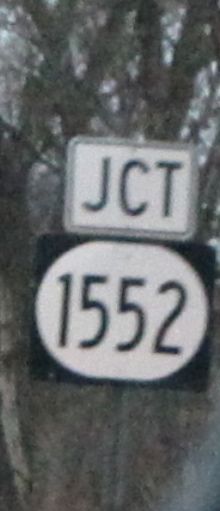This photograph captures a pair of road signs mounted on a single, likely steel, post situated against a hazy, blurred backdrop of trees, implying the setting is a rural or wooded area. The uppermost sign is a small, white rectangle outlined in black and bears the abbreviation "JCT," signifying the vicinity of an intersection with another route or highway. Below it, a larger, circular sign features a black background with a white border and displays the route number "1552" in prominent black numerals at its center. The image is vertically oriented, contributing to its tall and narrow appearance, and the overall scenery appears misty or cloudy, indicating it may have been snapped under conditions of limited visibility such as fog, mist, or rain. The photograph's grainy texture, combined with the indistinct details of the tree—suggesting it may be out of season or lacking foliage—adds to the atmospheric and somewhat enigmatic feel of the image.